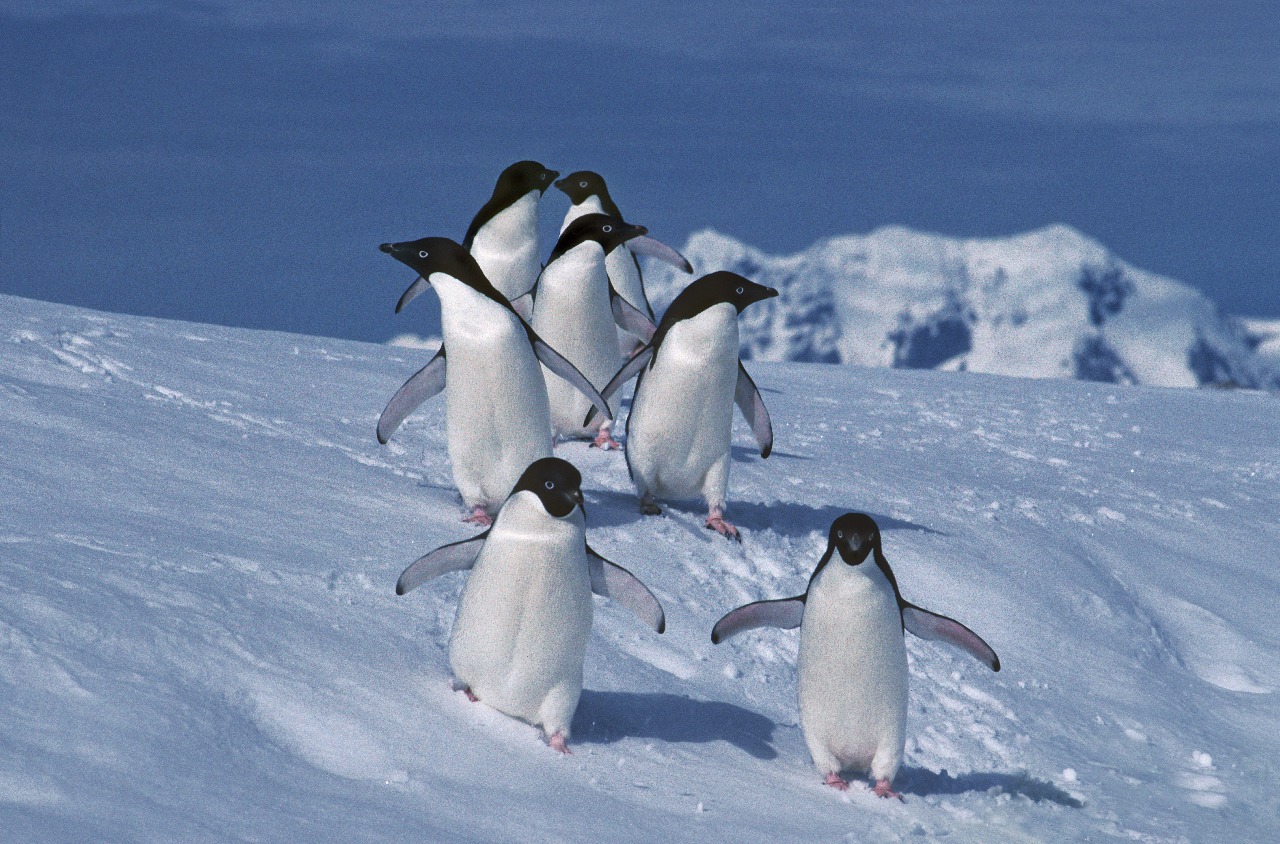This photograph depicts seven penguins walking down a snowy hill, angled towards the camera. Their formation is almost in pairs: two penguins are at the forefront, two slightly behind them, one in the middle, and two more penguins towards the back. The penguins have white bodies with black backs and heads, black beaks, and pinkish claws, with most spreading their wings as if balancing. The hill, covered entirely in white snow, slopes down towards the viewer, bisecting the image horizontally. There are numerous other penguin footprints visible in the snow, indicating heavy penguin activity in the area. In the background, the hill ascends to reveal a massive white glacier or a snow-capped mountain slightly to the right. Above, the sky or ocean appears in a dark blue shade, devoid of clouds, enhancing the chill and isolation of the scene.